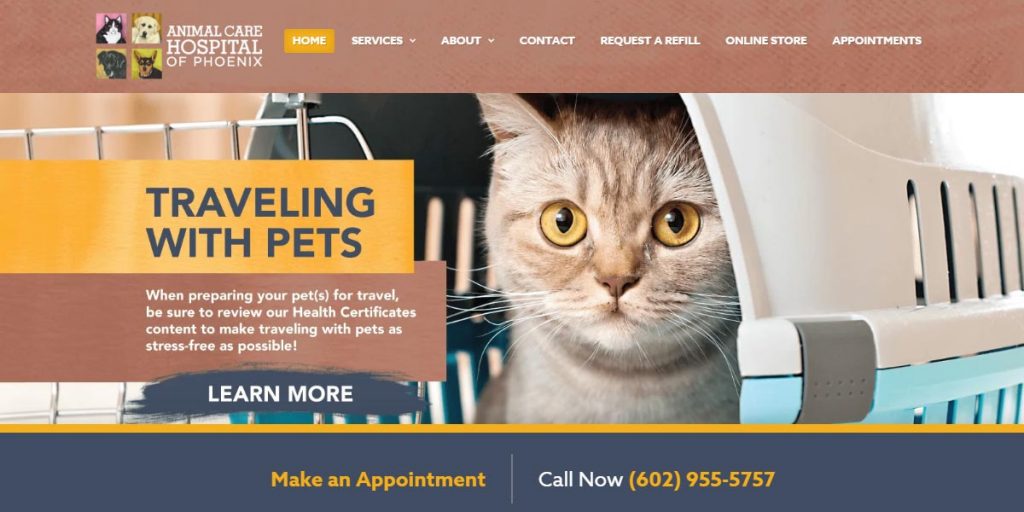At the Animal Care Hospital of Phoenix, an image showcases several pets: a white dog, a black dog, a black and white cat, and a brown and black dog. To the right of the image, there are navigation options labeled "Home," "Services," "About," "Contact," "Request a Refill," "Online Store," and "Appointments." Below these options, a brown and blue plastic animal carrier is featured. The carrier, held together by a gray clip, has a brown top and a blue bottom, with a metal gate that is open. Inside the carrier, a gray and white striped cat with large, bulging eyes and white whiskers is visible. A text section titled "Traveling with Pets" offers advice: "When preparing your pets for travel, be sure to review our health certificates content to make traveling with pets as stress-free as possible." Additional call-to-actions include "Learn More," "Make an Appointment," and "Call Now" with the phone number (602) 955-5757. The top of the text section features a brown border with white writing, while the bottom has a grayish-blue background with orange writing. The middle text incorporates shades of gray, blue, and white.